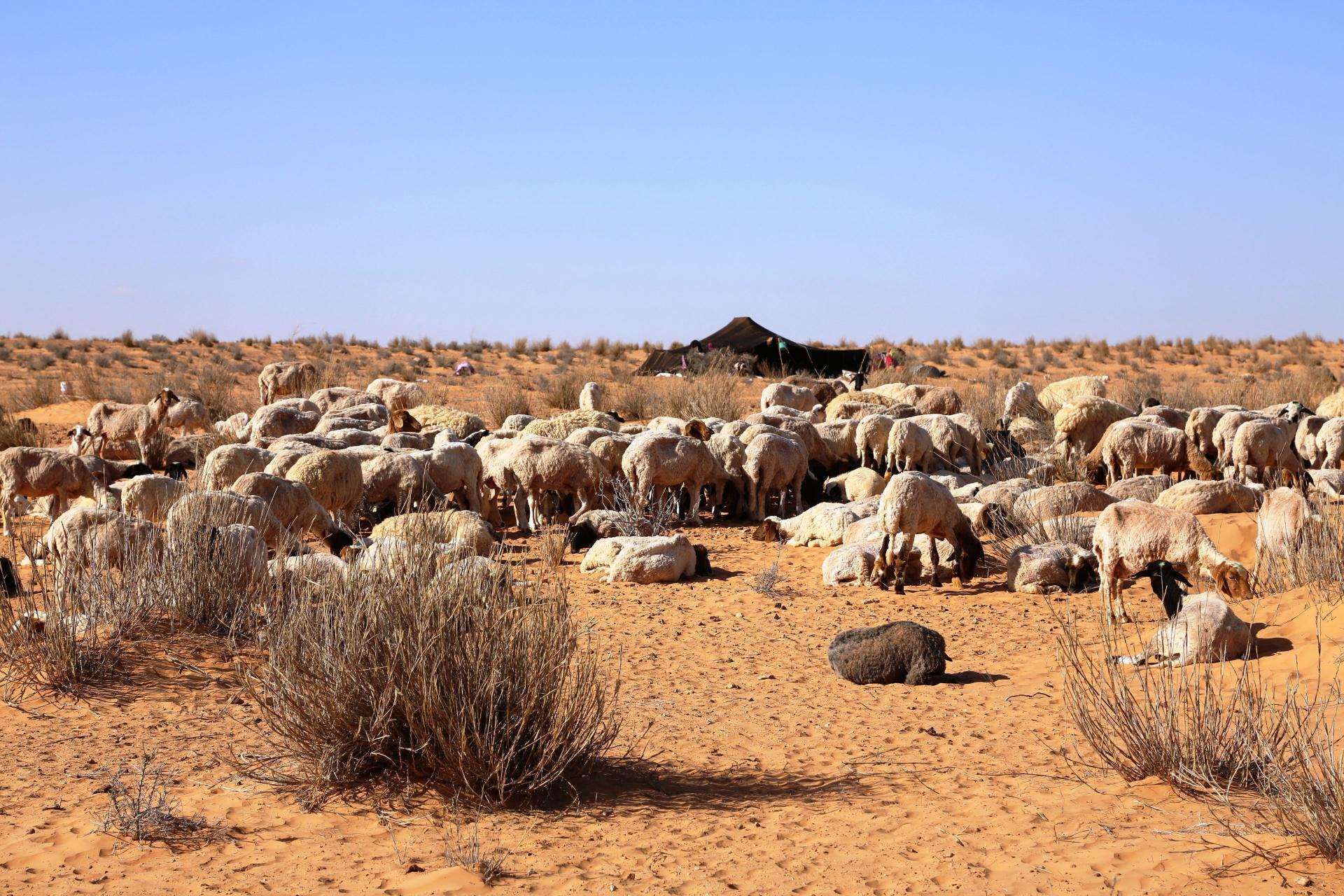In a vast high desert scene under a strikingly blue sky, we observe a large flock of around fifty sheep scattered across the arid landscape. The sheep are either leisurely grazing on the sparse vegetation or lying down for their midday rest amidst an expanse of dirt, dead bushes, tumbleweeds, and occasional rocks. Dominating the foreground is a black car surrounded by numerous people, creating a dynamic contrast to the serene pastoral activity. Behind the sheep, a sizeable tent with side flaps is pitched, likely providing shelter for the shepherd overseeing his flock as they forage. The expansive desert stretches towards the horizon, encapsulating the rugged beauty and tranquility of this picturesque rural tableau.